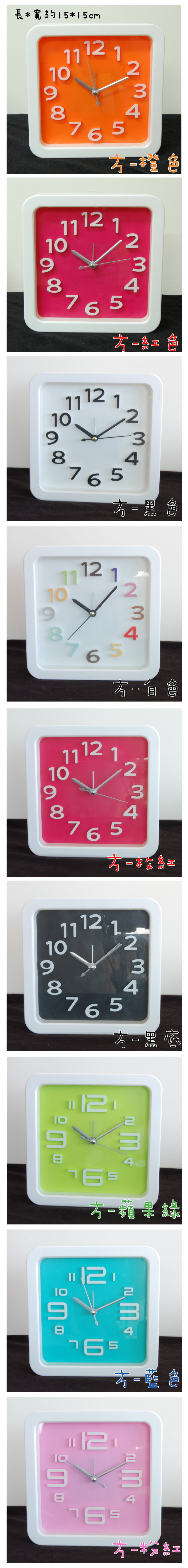This photograph displays a captivating montage of nine square alarm clocks arranged in a 3x3 grid pattern. Each clock, uniform in shape with a rectangular face and a defined white border, showcases a distinct color scheme. At the top, the clock features an orange face, with hard-to-read white numerals and gleaming gold hands. The second clock down boasts a pink background with crisp white numbers and hands. The third clock in the vertical series presents a classic white face accented by black hands and numerals. The fourth clock breaks the pattern slightly with a combination of black and red numbers paired with black hands. Midway down, a hot pink face with contrasting white numbers and hands draws attention. The sixth clock exhibits a bold black face, punctuated by white hands and numerals. Following this, the seventh clock stands out with a vivid lime green face, dark green hands, and white numerals. The eighth timepiece shows an aqua blue face with harmonious gray hands and white numerals. Completing the ensemble, the ninth clock situates a light pink face with gray hands and white numerals at the bottom of the array. Each clock's unique coloration and design contribute to a visually stimulating and artistically cohesive display.